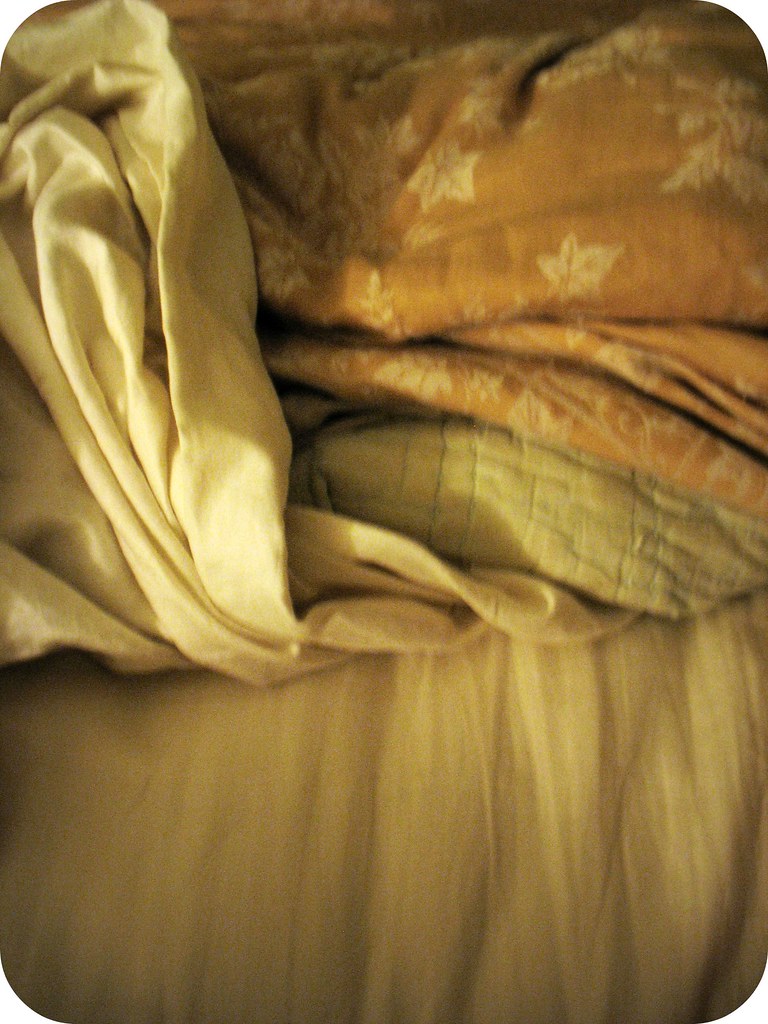A crumpled arrangement of textiles is displayed in this photograph, possibly taken on a bed or sofa, though the exact location is unclear. Notably, the image features no people, text, or date. Dominating the composition is a gold comforter adorned with cream-colored leaves, appearing slightly crinkled and displaced as if someone recently sat in the middle. Underneath, there is a contrast of layers: a lighter gold sheet, and a thicker, plain white blanket with visible stitching. The lower section reveals an additional white cloth, standing upright amidst the folds, hinting at the disordered nature of the setup. The overall scene is bathed in a warm light, reinforcing the slightly disheveled yet cozy aesthetic captured within the frame.